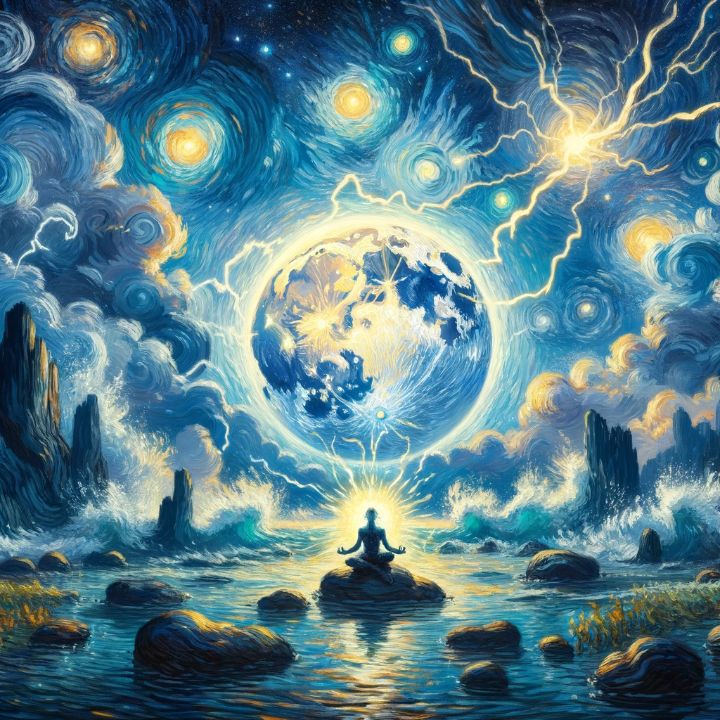This detailed painting, reminiscent of a Vincent van Gogh style, predominantly features blue, yellow, green, and brown hues. The scene centers around a person sitting cross-legged in a yoga or meditative pose, with arms extended and palms facing upward, positioned on a rock protruding from a body of water. The individual's head is tilted upwards, and they are enveloped in a glowing yellow light. Above them, a large celestial body—possibly a planet or moon—dominates the sky, surrounded by swirling clouds and large yellow orbs that resemble stars. Rock formations and mountains frame the sides of the image, contributing to the painting's serene and mystical atmosphere. The absence of text directs all focus to the tranquil and contemplative scene depicted.